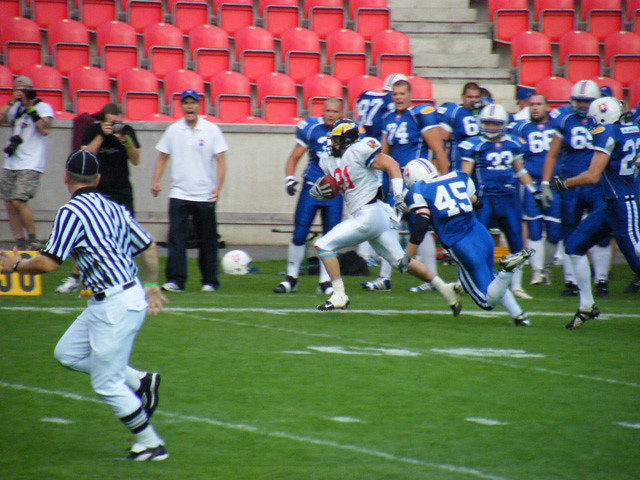In the midst of a high-energy football game, a player wearing a blue and yellow helmet, a white uniform displaying the number 21 in red, is sprinting down the vibrant green field, clutching the football firmly in his right hand. The environment is indicative of either a collegiate or NFL level competition, discernible by the apparent age and physique of the athletes. The scene unfolds within a vast stadium, though the empty red seats in the background suggest a sparse crowd or possibly a mid-game moment. 

On the left side of the image, two photographers are diligently capturing the unfolding action, while a referee clad in the traditional black and white striped shirt paired with white pants, is caught in motion at the corner of the frame. On the sideline, a coach can be seen animatedly shouting directions or encouragement to the players.

In hot pursuit of the ball carrier is an opposing player, number 45, donning an all-blue uniform and a white helmet. Meanwhile, other players from both teams are beginning to react, their movements indicating they are gathering around the right-hand side of the frame to engage in the play. This dynamic and detailed scene encapsulates the intensity and excitement of the game in progress.